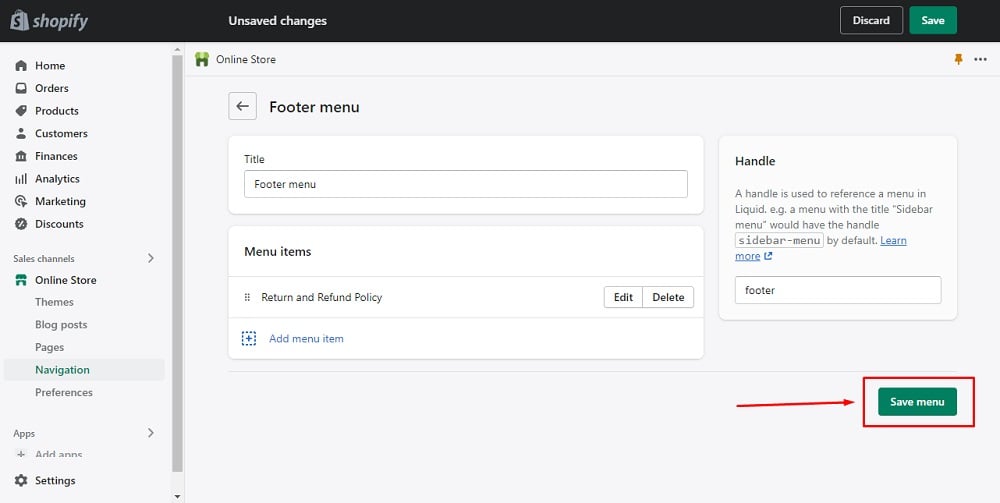In the image, we see a user interface of a Shopify dashboard with a very light blue background. At the top of the interface, there is a black notification box. On the left side of this box, there is a small shopping bag icon adorned with a dollar sign, indicating Shopify. The text "Shopify" is displayed prominently next to it, accompanied by the message "unsaved changes." To the right within the same box, there are two buttons: a black "Discard" button and a green "Save" button.

On the left side of the light blue background, there is a vertical navigation menu that includes the following options: Home, Orders, Products, Customers, Finances, Analytics, Marketing, Discounts, and Sales Channels. Each menu item has an accompanying rightward arrow, indicating sub-menus or expandable options. The "Online Store" and "Navigation" options are highlighted.

Towards the right side of the interface, there is a vertical blue slide bar. To the right of this bar, there is a section labeled "Online Store" which features a small green icon resembling an "H". Next to this, there is a red tag with three small dots.

Beneath this, a section displays a footer menu on a white background. It includes a title "Footer Menu" with subsequent fields for "Menu Items" and a "Return and Refund Policy." Each item has "Edit" and "Delete" buttons next to them. Additionally, a small blue square icon accompanies an "Add Menu Item" option.

On the right side of the interface, there is another light blue box titled "Handle." This section explains that a handle is used to reference a menu in Liquid, providing an example with the sidebar menu. It includes a default handle: "sidebar-menu" and a "Learn more" link in blue with an arrow.

At the bottom of the interface, there is a notable red arrow pointing towards a red outline around a green "Save Menu" button, emphasizing its importance for saving changes made to the menu settings.